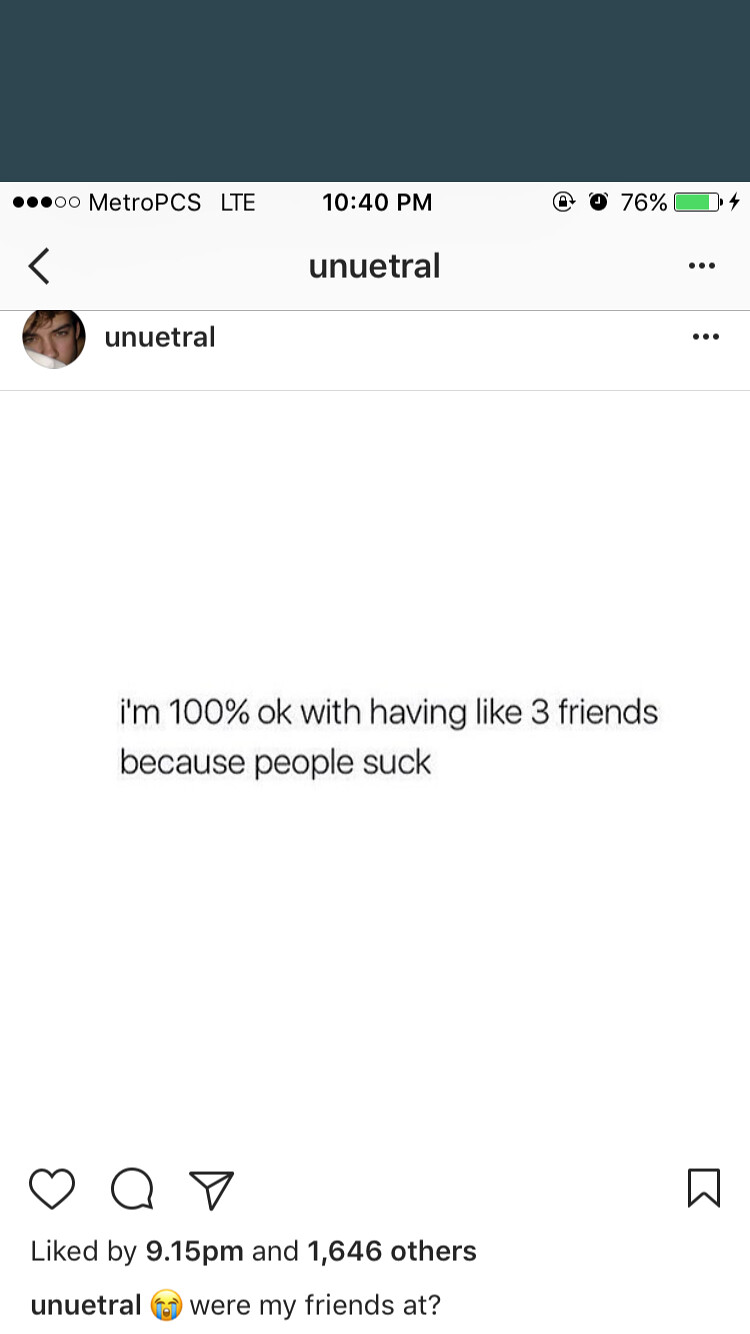The image is a detailed screenshot of a Metro PCS LTE phone at 10:40 PM, with 76% battery life indicated by a green, mostly filled battery icon with a small plus sign. The signal shows three bars. The upper-right corner features the name "UNEUTRAL" alongside a profile picture of a Caucasian male. The primary content is a meme that reads in black digital ink, "I'm 100% okay with having like three friends because people suck." The post has interaction icons below it, including a heart, a speech bubble, a paper airplane, and a bookmark. It shows it was liked by "9:15 PM and 1,646 others." UNEUTRAL commented with a laughing emoji, "where my friends at?" missing the 'E' from "where." The entire background is white.